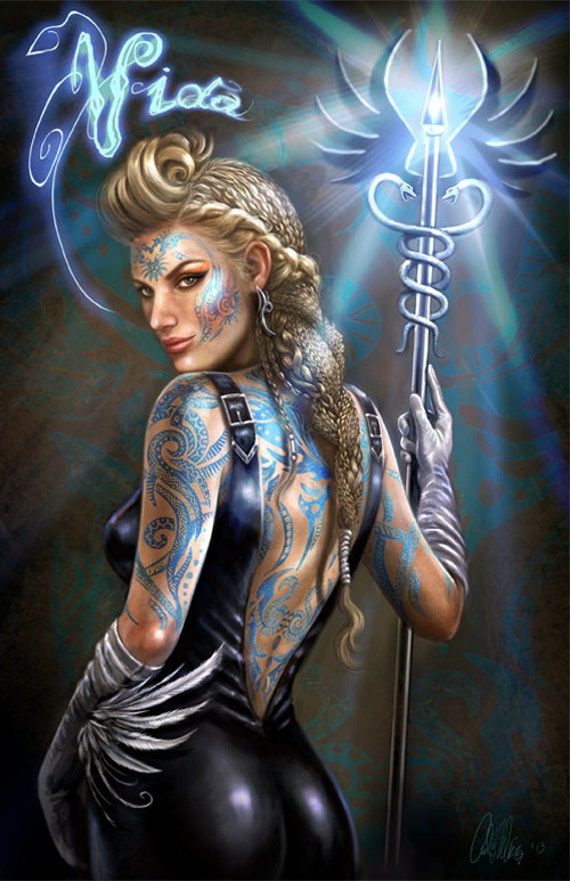This is a detailed hand-drawn illustration of a mythical female character, likely from a fantasy story or video game. The image showcases a woman with her back to the viewer, dressed in a tight, open-back black leather bodysuit accentuated with numerous blue tattoos resembling snakes and flowers on her face, back, and arms. Her long, braided golden hair features a prominent curl in the front, reminiscent of a large, rolled-back bang. She wears decorative silver gloves or armlets that look like short wings. In her right hand, she holds a staff adorned with twin snakes and spikes, emitting a blue glow at the top that forms the shape of a star. Above her head, in light blue neon script, her name is written as Vida, styled as if drawn by a fairy's finger in the sky. She appears to be smizing, with a wisp of smoke emanating from her mouth adding to her mystical aura.